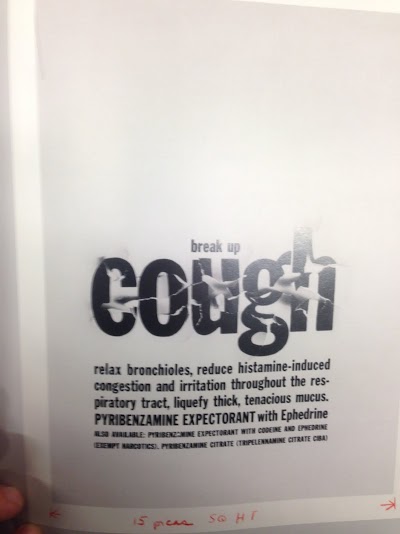This image appears to be a proof or mock-up of a magazine advertisement displayed on a gray background with a white border on the left and right sides. At the bottom left, a pair of fingers is holding or positioning the page for the camera. The main text on the page is in black, reading "BREAK UP" in smaller letters at the center, followed by the larger and more stylized word "COUGH," spelled out as C-O-U-G-H with jagged lines resembling mucus dripping from the letters. Below this, detailed text describes the product's function: "Relax bronchioles, reduce histamine-induced congestion and irritation throughout the respiratory tract, liquefy thick, tenacious mucus." The advertisement names the product, "Pyribenzamine expectorant with ephedrine," and mentions an alternative version containing codeine and exempt narcotics. In very fine print at the bottom, there is a list of chemical ingredients. Additionally, handwritten text in red can be seen below the detailed text, suggesting editorial notes or further instructions. Overall, the ad evokes a clinical and somewhat unappealing visual portrayal of mucus to emphasize the product's utility.